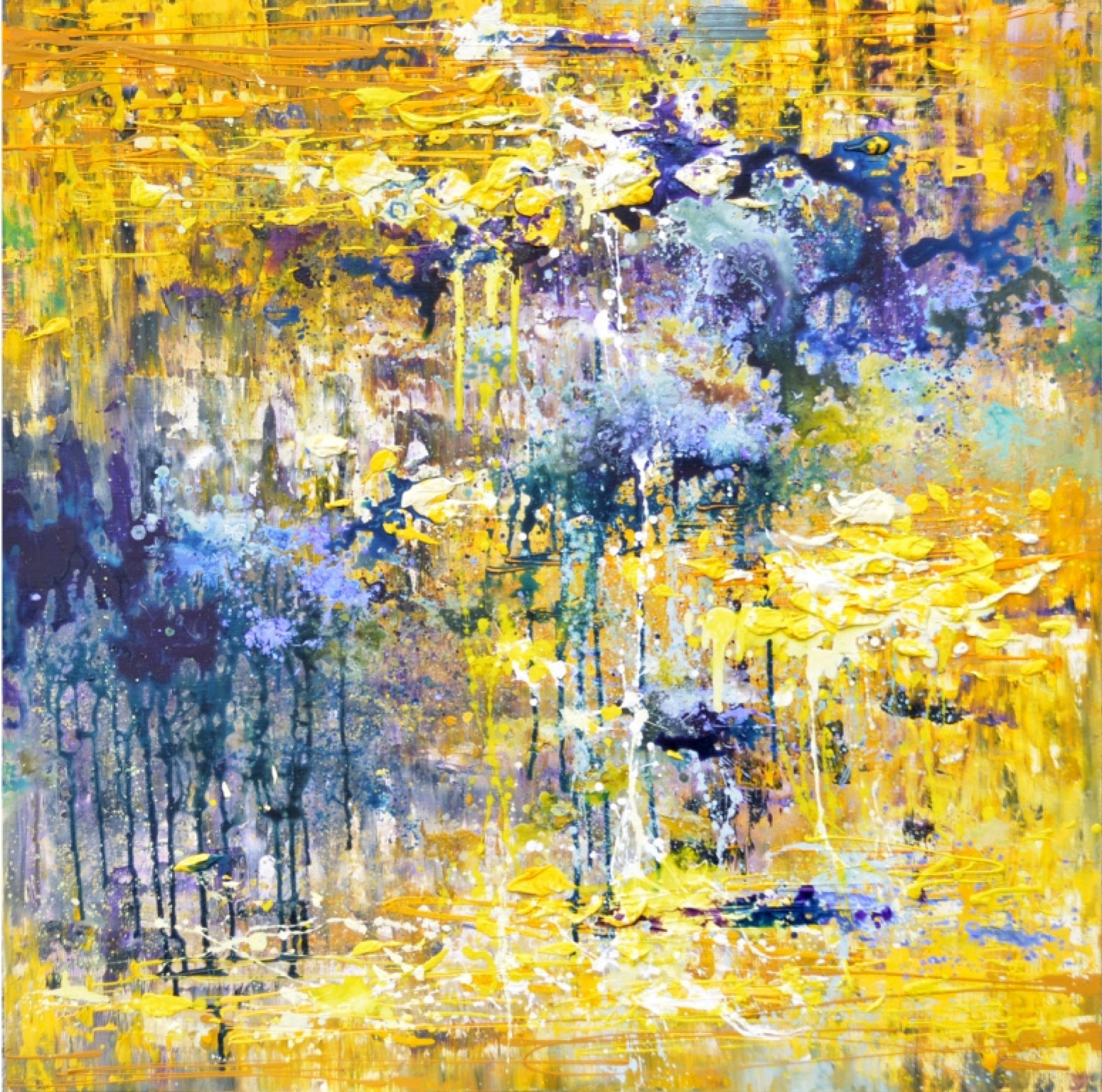This detailed abstract oil painting bears resemblance to Monet’s Water Lilies, capturing a reflective scene in a still pond. Predominantly showcasing a vivid yellow and blue color palette, the painting features a rich texture achieved through the layered brush strokes that create a piled effect of paint. In the lower left, bright blue spots suggest the presence of water or flowers, while clumped yellow patches evoke a sense of sunlight. The scene appears to depict reflections of land and trees, with blue tree-like structures standing vertically towards the center. The painting transitions from yellow and white hues at the bottom to mixed blue and white vertically, culminating in a predominantly yellow and white upper section. The top left corner exhibits hints of orange lines, contrasted by darker blue shades on the right, enhancing the overall dynamic movement within the abstract portrayal of the serene pond.